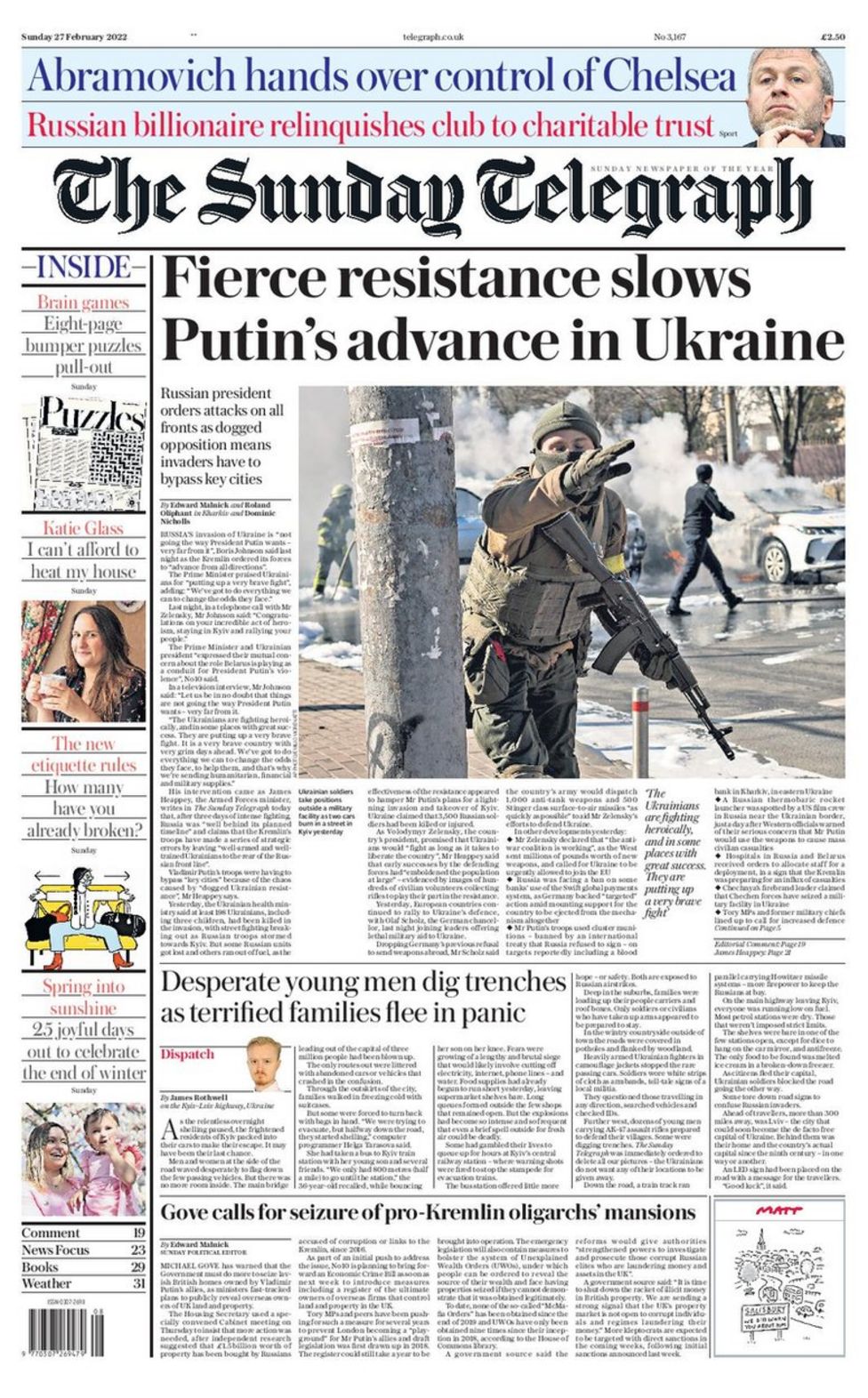**Caption:**

Under the category "Website," this image highlights the front page of The Sunday Telegraph. The headline announces "Abramovich hands over control of Chelsea," followed by subheadings: "Russian billionaire relinquishes club to charitable trust." At the top, bold and ornate letters spell out "The Sunday Telegraph." The main story, titled "Fierce resistance slows Putin's advance in Ukraine," is accompanied by a vivid photograph. In the foreground, a soldier carrying a rifle is prominently visible. Behind him, a person crosses the street while firemen work to extinguish fires in the background, where a car is seen emitting smoke near a telephone pole. Additional articles include "Desperate young men dig trenches as terrified families flee in panic" and "Gove calls for seizure of pro-Kremlin oligarchs' mansions." In the top left corner, a section marked "Puzzles" features a display of crossword puzzles.